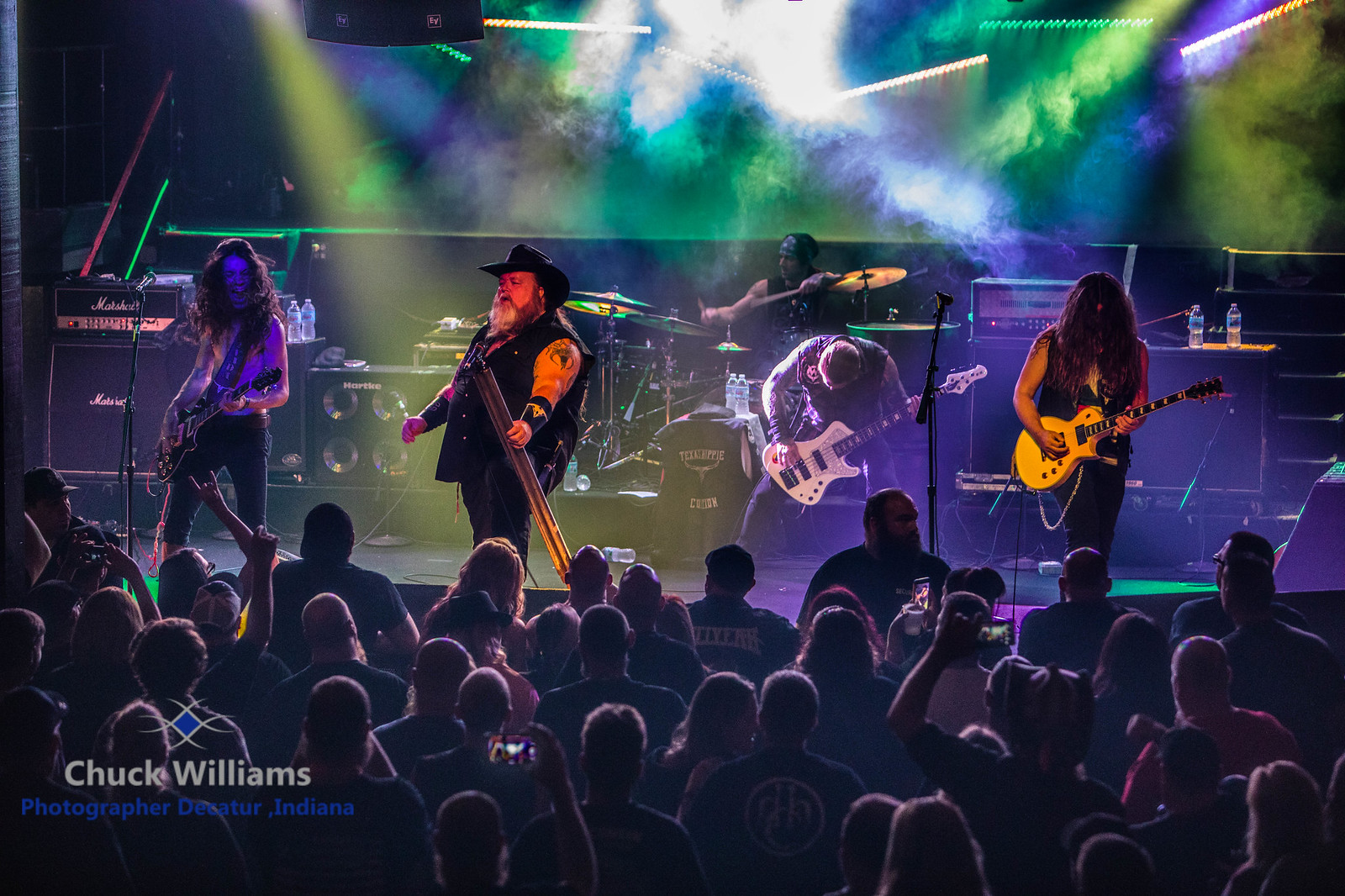The photograph captures the electrifying atmosphere of a rock concert, viewed from the audience's perspective. The stage is bathed in vibrant green, blue, yellow, and white lights, contrasting sharply with the darker crowd. The audience, a sea of heads and shoulders, faces towards the stage, some holding up phones and cameras to capture the moment.

Central to the scene is the band, featuring five members. The lead singer, a heavyset man with a beard, dons a black cowboy hat, a sleeveless black button vest, and black pants. He wields a microphone, engaging the crowd. To his left is a shirtless guitarist, also clad in black pants, with long hair cascading down as he energetically screams into the audience, his black electric guitar grasped firmly. 

On the singer’s right stands another guitarist, headbanging with a white guitar, dressed in a black vest with long hair flowing. Next to him is a third guitarist, similarly adorned in black, playing a white guitar. Behind the frontmen, the drummer is visible with a dark-colored drum kit, sporting a bandana and a cut-off sleeve t-shirt.

The stage is adorned with standard speakers, water bottles, and artistic lights. A Marshall amplifier is noticeable behind the shirtless guitarist. An event staff member is seen near the stage, providing an added layer of security alongside what appears to be a bodyguard between the guitarists on the right. The photograph credits “Chuck Williams” as the photographer, potentially from Decatur, Indiana. The overall composition vividly encapsulates the dynamic and vibrant essence of a live rock concert.